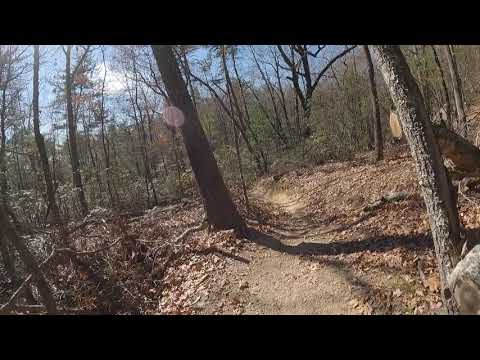The image captures a serene forest setting with a narrow dirt path winding through the woods. It suggests a snapshot taken perhaps in autumn or early spring, as the trees are mostly bare, and the ground is strewn with dead leaves, twigs, and rocks. The trail is barely wide enough for a single person and appears slightly overgrown, sloping into a ditch to the left. Imposing tree trunks dominate the scenery, with one notable dark brown tree leaning heavily to the left and a light grayish trunk drawing attention on the right. On the right side of the path lies a decaying fallen log amidst a forest floor of dead leaves and debris. The background features possible evergreen trees and various shades of green foliage, although some details remain indistinct. It's a bright, sunny day with a light blue sky punctuated by a single fluffy white cloud. The image is framed by black strips at the top and bottom, enhancing the natural, unprofessional quality of the photograph. The overall palette includes blacks, browns, yellows, grays, shades of blue, and some rusty orange, reflecting the transition of seasons.